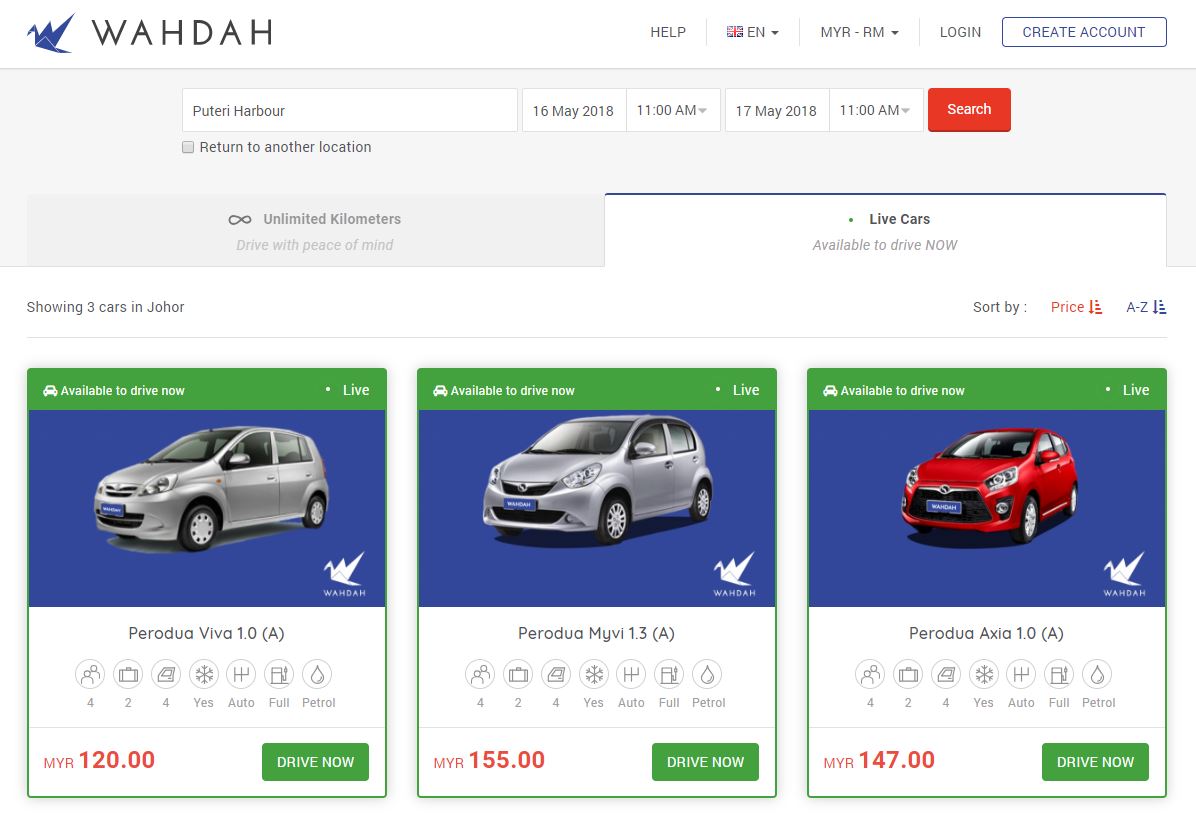The image depicts a web page interface, primarily characterized by a clean, white background. In the upper left-hand corner, there is a blue origami swan next to the title "Wada," serving as the logo. Below the logo, there is a search functionality tailored for finding available cars to drive immediately. This search section is followed by three boxes, each showcasing a different SUV model. The first two boxes display silver-gray SUVs, priced at $120 and $155 respectively, while the third box features a red SUV priced at $147. Each car listing includes a green button labeled "Drive Now," inviting users to initiate the driving process. Color elements on the page include accents of blue, green, and red, providing a vibrant contrast to the white background.